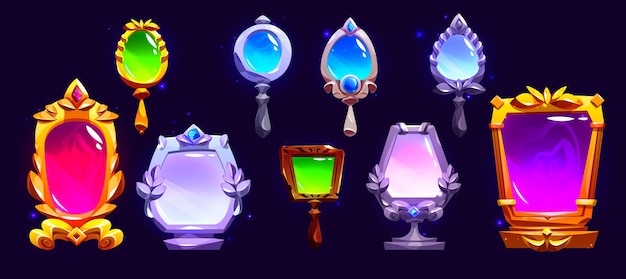This is a highly detailed digital rendering set against a black background, depicting an assortment of ornate mirrors rather than jewels. The composition includes nine distinct mirrors, each with unique shapes and color schemes. In the top row, there are handheld mirrors: the first on the far left is gold with green glass, followed by another with a purple handle and blue glass. The third is diamond-shaped, pink with blue glass, and the fourth is purple and triangular, also featuring blue glass. In the bottom row, there are larger standing mirrors, starting with a gold one housing pink glass. Another standing mirror is purple with purple glass, alongside a handheld mirror designed to resemble wood with green glass. Adjacent is a purple standing mirror with pink glass, and finally, a gold standing mirror with purple-pink glass. The image lacks descriptive text, leaving viewers to appreciate the artistic representation of these varied and colorful mirrors, which some might initially mistake for jewels.